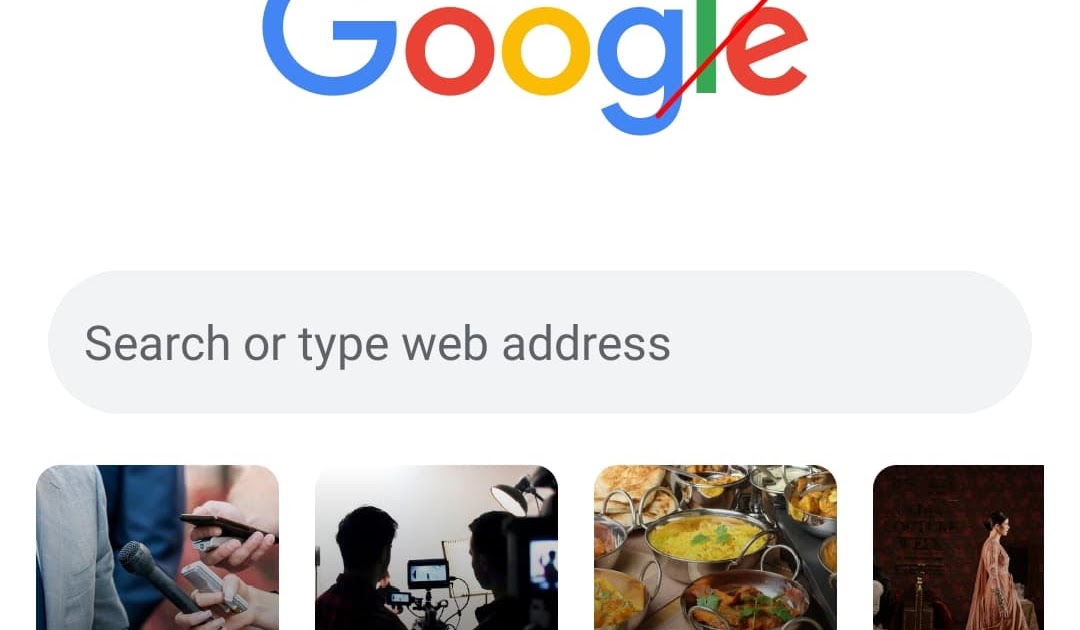The image displays the Google logo, partially cropped at the top, cutting through the upper segment of the letter 'C', part of the first 'G', and 'L'. The logo features the characteristic Google colors: the first 'G' is blue, the first 'O' is red, the second 'O' is yellow, the second 'G' is blue, the 'L' is green, and the 'E' is red. A vibrant red diagonal line slashes through the logo, beginning at the top of the 'E', cutting across the 'L', and intersecting with part of the 'G'. Surrounding this scene is a field of white space that transitions into a gray oval containing inscribed text. The message reads "Search with a capital S or type web address" in black font.

Below this, there are four distinct images aligned in a row. The first image on the left features a microphone, two recorders, and a phone. The devices are positioned in front of a gray suit jacket, though no person is visible. The second image shows two people looking at cameras, with a third individual positioned in front of the camera, all set against a stark white background. The third image depicts a food platter with various bowls containing food items in colors such as yellow, green, brown, and beige, though the specific foods are indiscernible. The final image showcases a model dressed in traditional Indian attire.